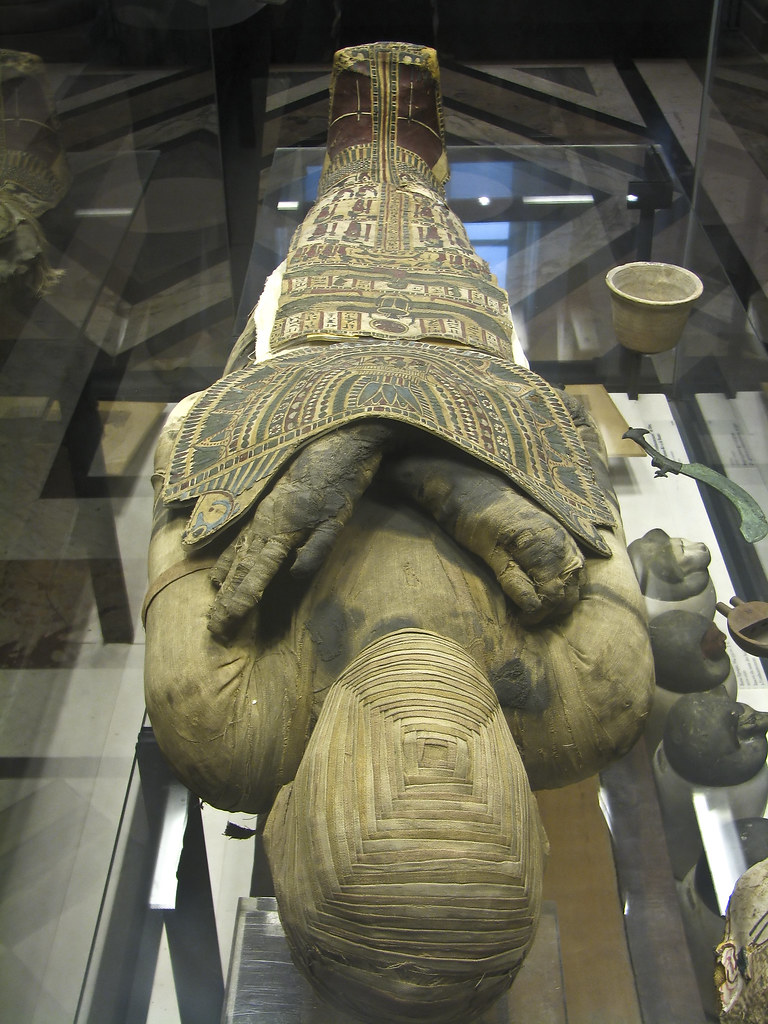This photo features an intricately-designed sarcophagus, traditionally used for Egyptian mummies. The head portion is situated at the bottom of the image, while the feet are at the top. The headpiece of the sarcophagus is made of metal and features a series of concentric squares, creating a captivating geometric pattern. The chest area, rendered in a light brown hue, includes detailed coverings for the shoulders. 

The arms of the sarcophagus extend down to its sides before crossing over the chest just below the shoulders, around the armpit area. This section exhibits a light tan and green coloration with dark black spots. Covering the arms is a flexible, shield-like metal material, predominantly gold and green. A similar material, characterized by gold, yellow, and red tones, covers the legs. 

The feet are enclosed in an iron casing with gold edges and red outlines, complemented by a central gold design. The sarcophagus rests in a glass case with a floor patterned in black, white, blue, and brown triangles. Additional details include a faint reflection of the feet on the left side and a small light brown cup at the waist level on the right side of the image.